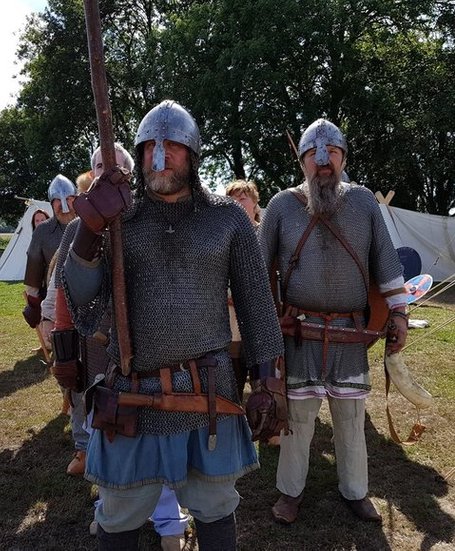The photograph depicts a vivid scene from a medieval reenactment or renaissance fair, set on a sunny summer day. In the foreground, several men are clad in elaborate chainmail costumes, with metallic silver helmets that shimmer in the bright light. The individual closest to the camera wears a blue kilt paired with modern-looking pants and sturdy, heavy boots. He grips a long handle that could either be a spear or the base of a banner pole, adding a touch of historical authenticity.

The background reveals a sprawling outdoor area with leafy trees, hinting at the warm season. Beat-up grass and patches of mud suggest frequent activity and foot traffic on the hill where the reenactment is taking place. White fabric tents dot the landscape, further emphasizing the medieval atmosphere. There are additional figures in the distance; some are dressed similarly in chainmail and armor, while others appear to wear civilian clothing, possibly spectators or family members mingling with the participants. Notably, one reenactor brandishes a large tusk likely used as a horn, enhancing the historical tableau. The scene is bustling with activity, capturing the essence of a large gathering dedicated to reliving and celebrating medieval history.